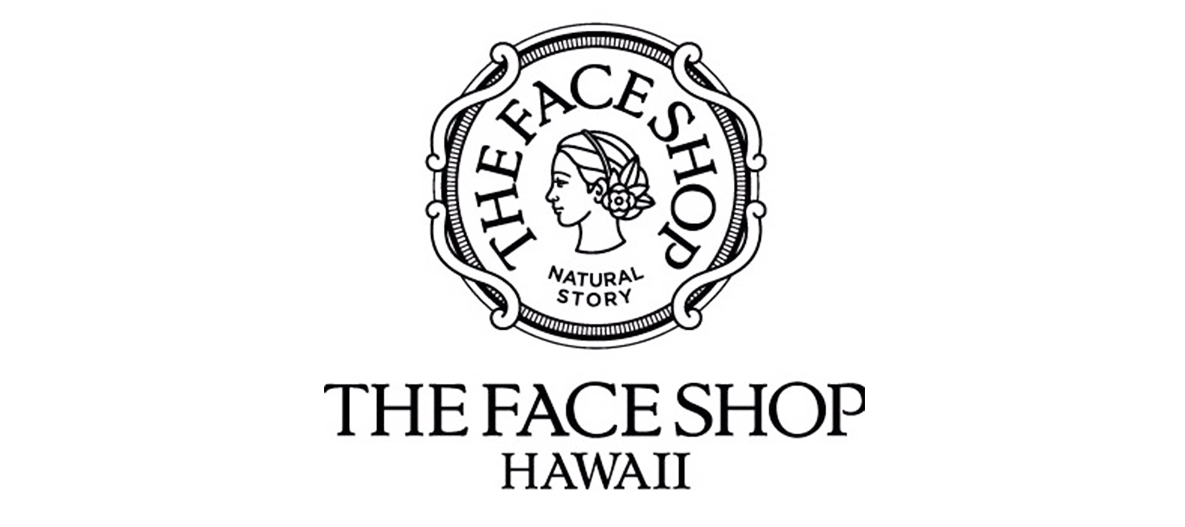The image depicts a black and white advertisement for The Face Shop, a business with a specific focus in Hawaii. Central to the image is a circular logo designed to resemble the intricate grooves of a coin. Inside this circular emblem, at its center, is the profile of a woman's head adorned with a headband and a flower positioned over her bun, giving a distinct tropical and natural feel. The text "The Face Shop" arches around the inside edge of the circle, accompanied by four delicate white swirls equally distributed. Below the circular logo, bold text reads "The Face Shop," followed by the words "Natural Story" and "Hawaii" in smaller font, emphasizing the store's natural product offerings and its Hawaiian connection.